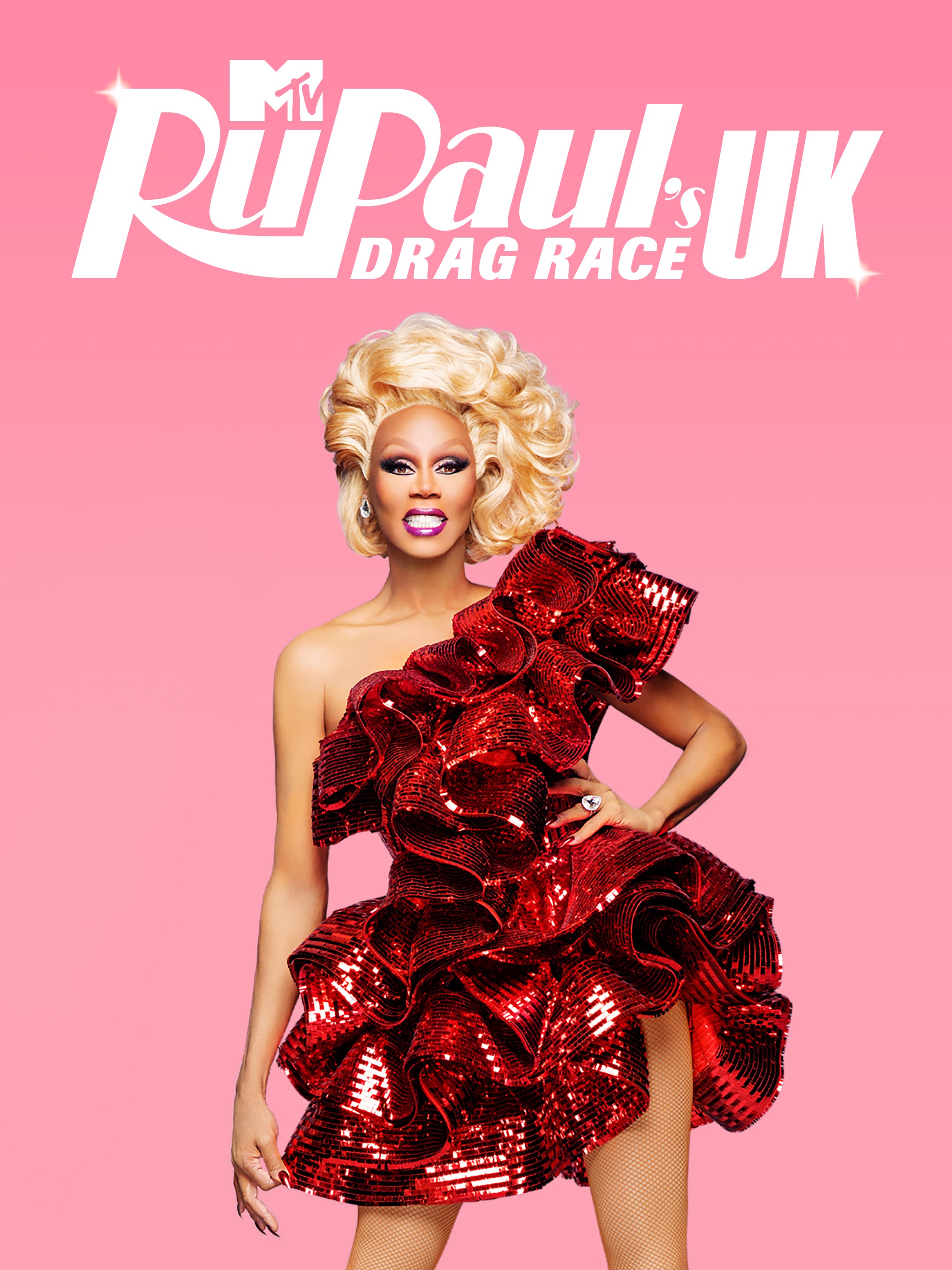This image is a promotional poster for MTV's "RuPaul's Drag Race UK." The entire background is a medium shade of pink. At the top of the poster, the MTV logo is displayed in white, followed by the show's title, "RuPaul's Drag Race UK," also in white lettering. Centered in the image is RuPaul, exuding elegance and glamour. RuPaul is dressed in a stunning, short, red sequined dress that is frilly and elaborate, featuring a one-shoulder design—one sleeve covers the left arm, leaving the right shoulder bare. Her blonde hair is styled high on her head with curls and swirls, adding to her dramatic look. Her makeup is bold, with dark eye makeup and purple lipstick accentuating her bright white smile. RuPaul's ensemble is completed with large diamond earrings and a distinctive ring on her left ring finger. Her nails are painted a bright red to match her dress. She is also wearing nude-colored fishnet stockings. RuPaul strikes a pose with her left hand on her hip, leaning slightly to the right, capturing the confident and glamorous essence of the show's spirit.